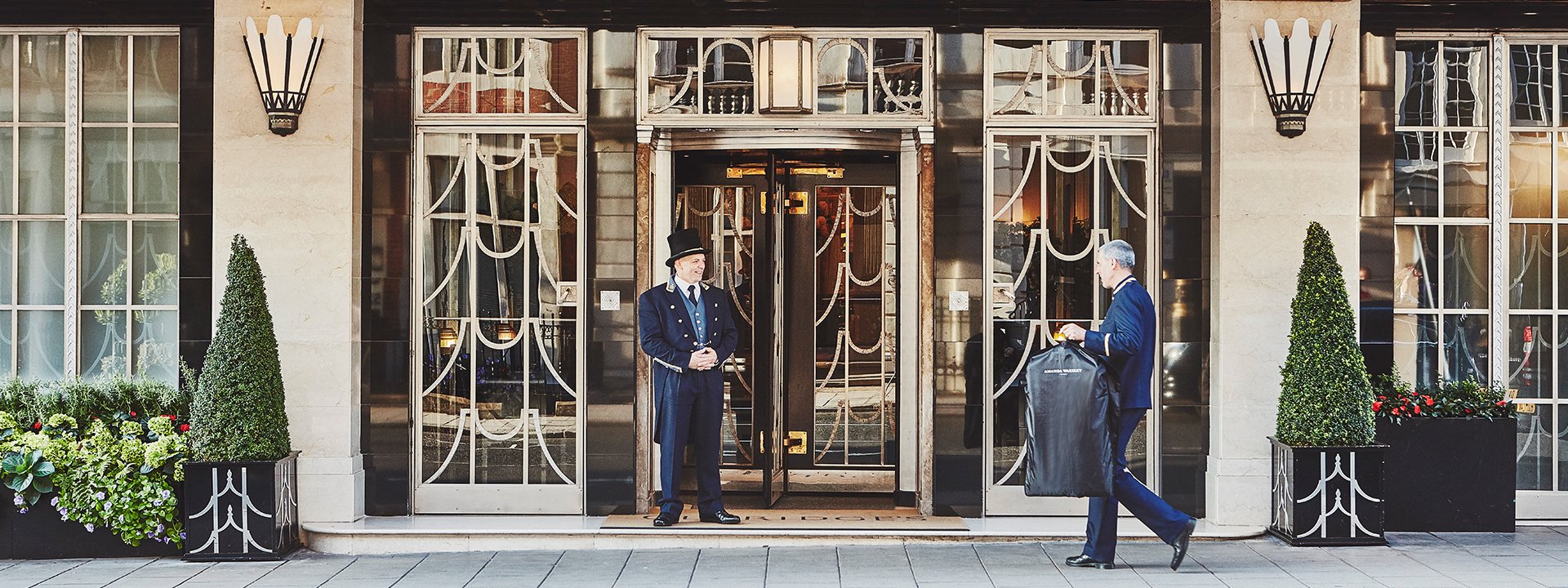In the photograph, we see two impeccably dressed gentlemen at the entrance of a lavish, stylish building that exudes an old-fashioned, grand hotel charm. The building features fancy patterned windows, glass doors, and large Art Deco style sconces adorning the entranceway. The man at the center, likely a bellboy or doorman, stands in front of a roundabout-style door. He’s wearing a black hat, a blue double-breasted coat with tails, a light blue vest, a black tie, a white shirt, matching dark blue pants, and black leather shoes. He is smiling at another man approaching from the right. This second gentleman is clad in a blue suit, carrying what appears to be freshly pressed clothes in a coat bag. Both men wear similar navy blue to dark purplish hues. Flanking the entrance are green Christmas tree-like shrubs placed in black square boxes with white patterns. The street lamps and lavish decor contribute to the building's luxurious and timeless aesthetic.